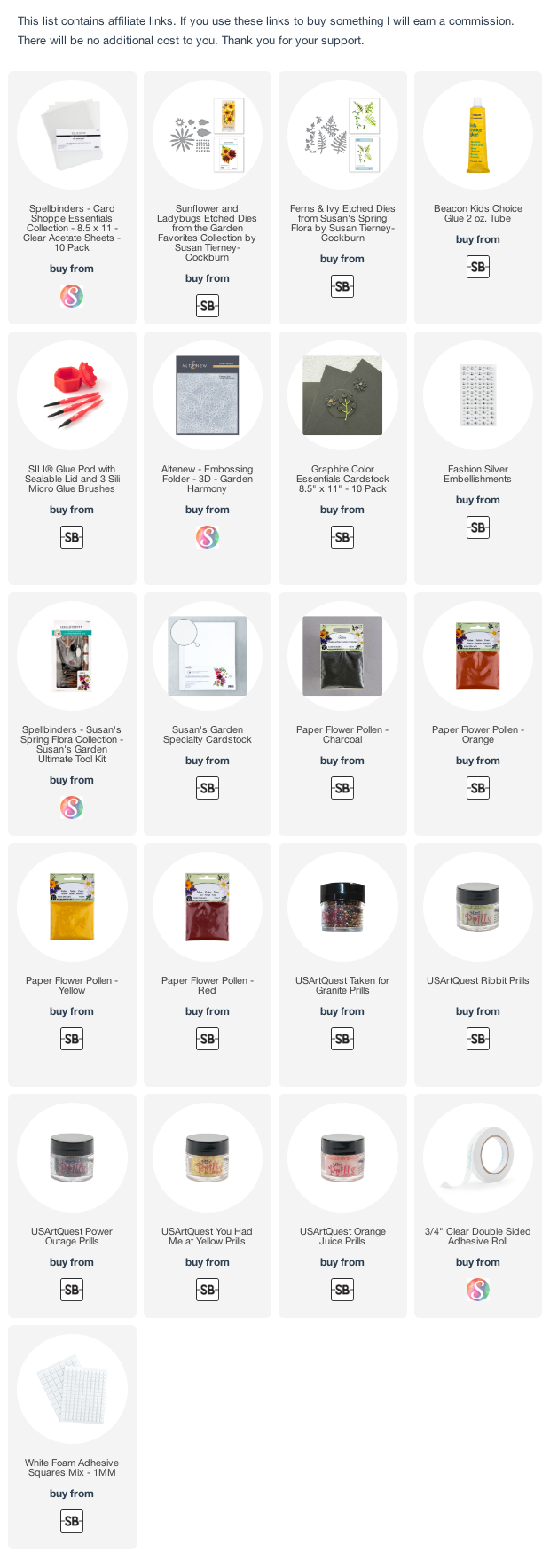An image of a shopping website displaying a diverse range of small-sized products neatly arranged in a grid format. The grid consists of four columns and five rows, with the exception of the first row, which includes six items. The products vary widely — some appear to be art supplies like paint tubes, while others resemble bedding items and containers of glitter with black lids. Additionally, there are items that look like rolls of sellotape. Each product is accompanied by a brief description, including the name and price, at the bottom of its respective image. The overall layout is compact, with many items tightly fitted onto the page, making them appear quite small.